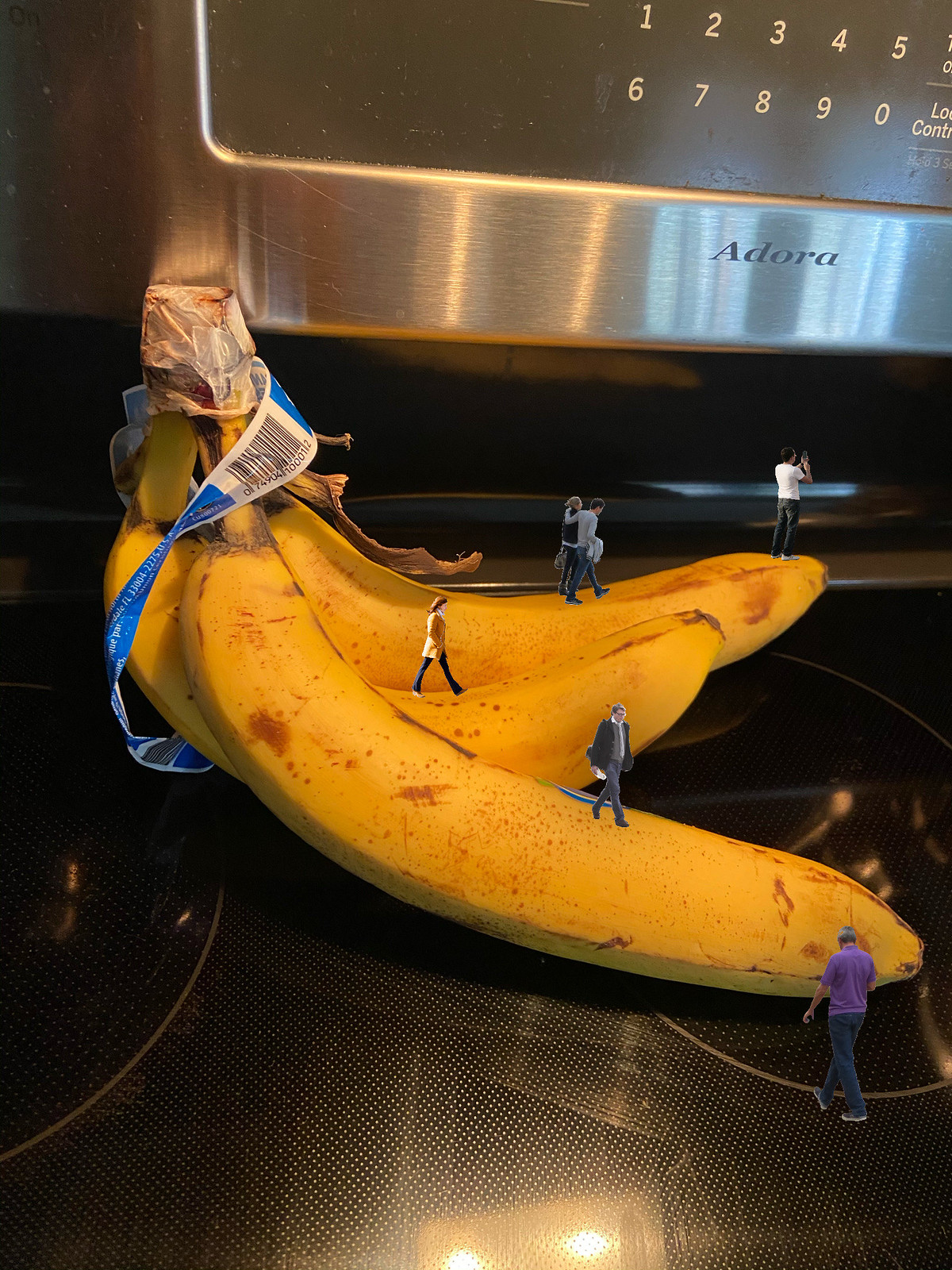This highly detailed and surreal image presents three half-ripened, yellow bananas with dark spots and a blue and white plastic label, including a barcode, centered on a sleek black electric stove surface. The stove, featuring the brand name Adora on a stainless steel display with controls numbered 0 through 9 and marked "low control," serves as a sharp, modern backdrop. Enhancing the whimsical nature of the scene, six miniature, colorfully dressed people are walking across the bananas as if embarking on a daily commute. Among them, a man and a woman share an intimate moment, arm in arm, adding a touch of human connection amidst the randomness. One solitary figure is also seen making their way on the black stove surface. This striking visual blends domestic familiarity with imaginative, miniature storytelling.